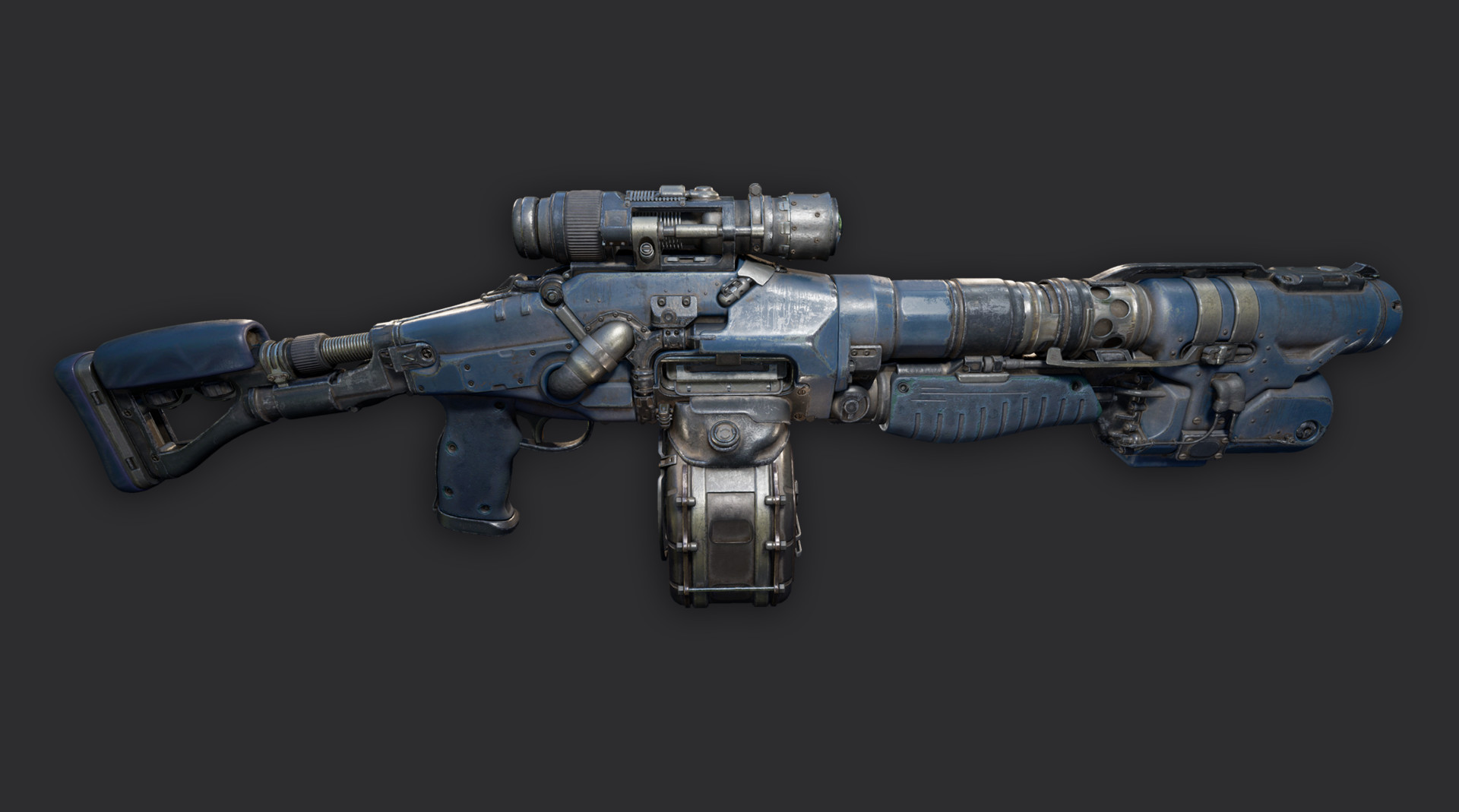The image portrays a futuristic, sci-fi inspired military-style machine gun suspended in mid-air against a dark charcoal gray backdrop. The weapon features an intricate design with a bluish-gray color scheme, accentuated by several exposed silver metal components that give it an industrial look. A prominent and bulky trigger stands out, indicating that it is built for significant power and rapid fire. The gun is equipped with a detailed scope mounted on top, positioned just above the pistol grip and trigger. The barrel, extending to the right, includes a large rubber grip and an expansive silencer, while the butt of the stock, located on the left, incorporates a spring mechanism to manage recoil. Additionally, the weapon showcases a drum magazine situated centrally and multiple chambers which could serve as extra ammunition storage. Various wires are seen interconnecting the components, possibly enhancing the gun’s power or functionality. Overall, the weapon's high-tech aesthetics and multiple advanced features suggest it could be from a futuristic war scenario or a sci-fi movie.